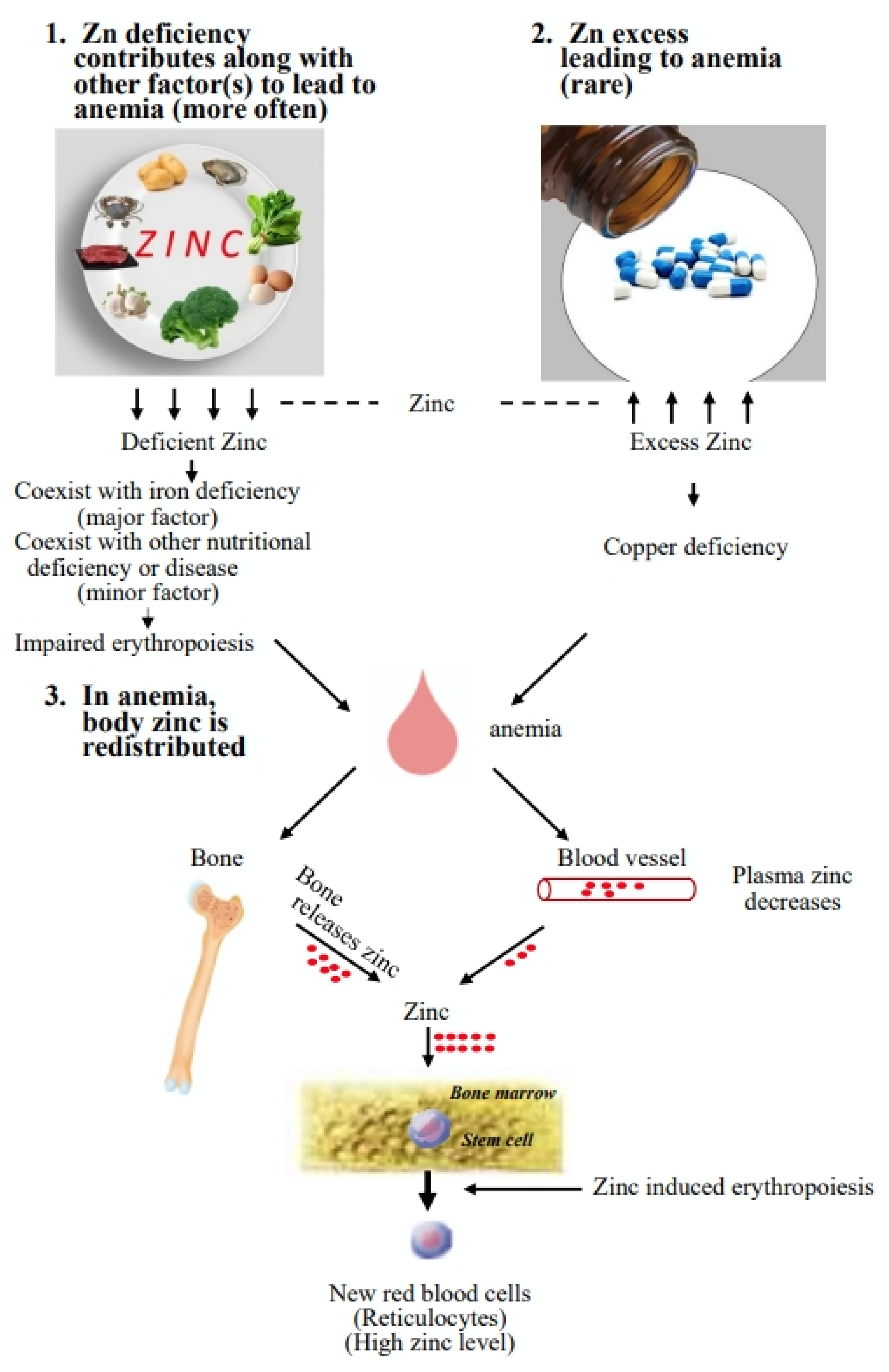This detailed diagram, set against a white background, illustrates the complex relationship between zinc levels and anemia. At the top left, the diagram explains that zinc deficiency, often accompanied by iron deficiency (major factor), other nutritional deficiencies, or diseases (minor factors), can lead to impaired erythropoiesis and subsequently anemia. This section is visually represented by a white dinner plate adorned with foods rich in zinc, such as broccoli, eggs, spinach, and crab, with arrows highlighting the progression from zinc deficiency to anemia.

To the top right, the diagram shows a less common scenario where zinc excess leads to anemia, depicted by a pill bottle spilling blue and white pills. This section explains that excessive zinc can cause copper deficiency, another pathway to anemia.

Connecting these concepts, the central part of the diagram describes the redistribution of zinc in the body during anemia. Arrows flow from a red blood droplet towards a bone and a blood vessel diagram, indicating a decrease in plasma zinc. Further arrows lead to bone marrow and stem cells, where erythropoiesis (production of red blood cells) is affected. The process concludes with the formation of new red blood cells with high zinc levels.

Overall, this comprehensive diagram effectively highlights the roles of zinc deficiency and excess, their interactions with other nutritional factors, and the resulting impact on anemia, providing a clear and concise visual representation of these biochemical relationships.